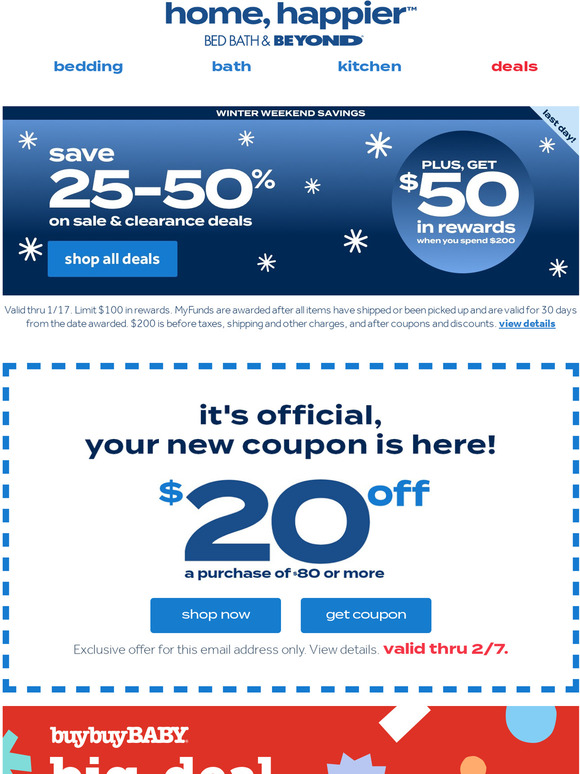**Screenshot of Bed Bath & Beyond Mobile Website**

The screenshot captures the mobile version of the Bed Bath & Beyond website, showcasing the brand's clean and user-friendly interface. At the top of the screen, the new slogan, "Home, Happier," is prominently displayed in bold blue font, followed immediately by the Bed Bath & Beyond logo.

Below the slogan, there are four clearly labeled drop-down menus for easy navigation through the website's core categories: Bedding, Bath, Kitchen, and Deals. This ensures users can quickly find the products they're interested in.

A central feature of the screenshot is a blue rectangle banner ad promoting a special sale. The banner announces substantial weekend savings of 25% to 50% off and highlights an additional incentive of a $50 reward. The banner is eye-catching and designed to capture the shopper's attention with its bright color and large font.

Underneath the banner ad, detailed fine print provides all necessary conditions and stipulations related to the sale and rewards, ensuring transparency and clarifying the terms for users.

Additionally, the screenshot includes a digital coupon that outlines various methods of utilization for shoppers. The coupon specifies the minimum purchase requirements needed for redemption, reflecting the typical conditions often associated with promotional offers on retail websites.

Overall, this detailed layout of the Bed Bath & Beyond mobile website emphasizes both usability and promotional offers, enhancing the overall shopping experience for users.